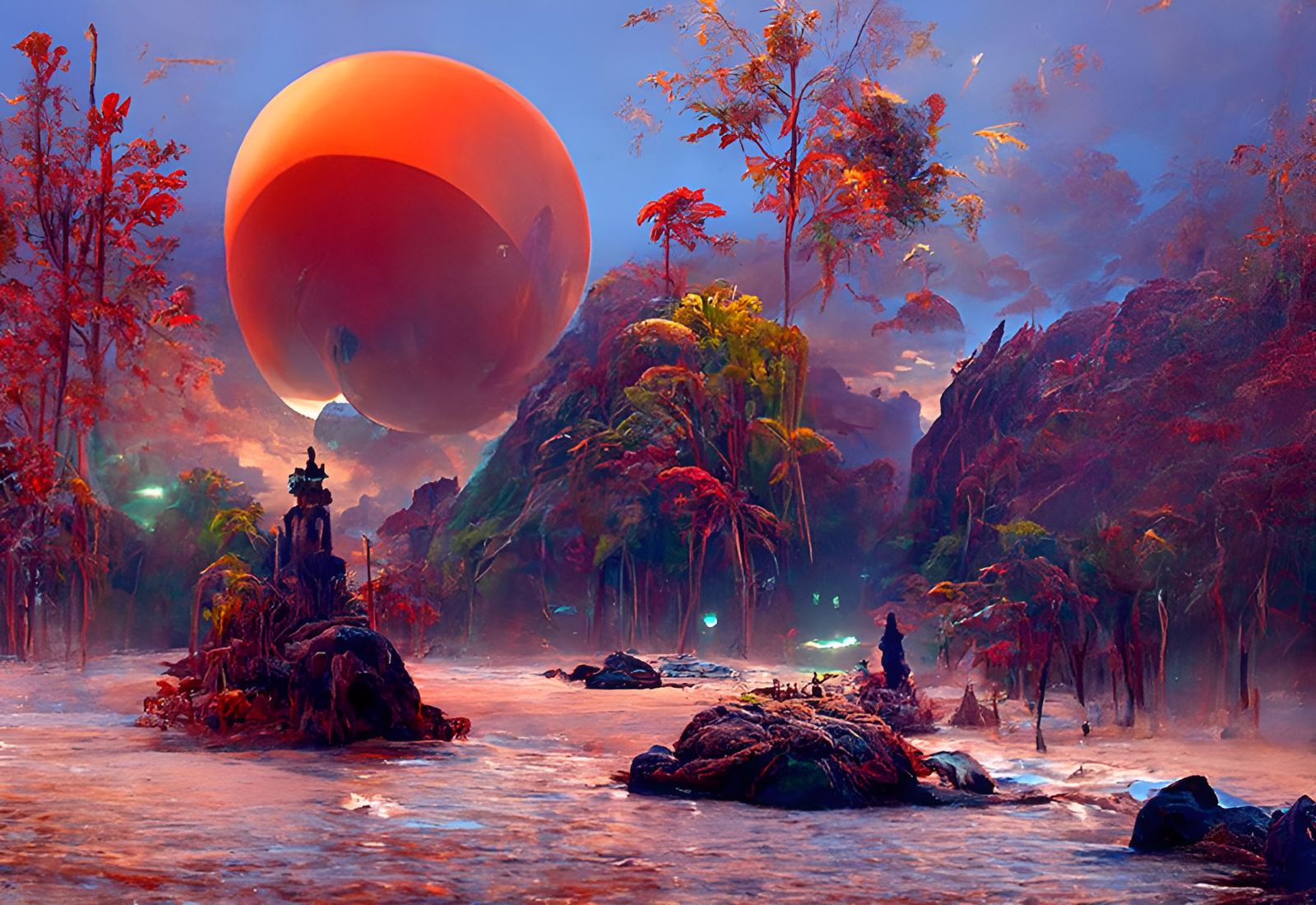The image depicts a fascinating and surreal nighttime landscape under a dark, eerie blue sky with occasional clouds. The scene is dominated by a large, enigmatic red-orange sphere or blob, occupying the upper left corner and extending towards the top of the picture. This mysterious object has varying shades of orange, adding to its indistinct and ambiguous nature. To the right and in the middle, a range of small, colorful mountains in striking fall colors—reds, oranges, and yellows—create a picturesque and vivid setting. 

On the left side, a cluster of red-orange trees complements the autumn palette. Near the front, a creek or river dotted with rocks flows gently, reflecting the moonlit sky. One of the rocks appears to have a person standing on it, adding a human element to this otherwise otherworldly scene. Central to the image are black structures seated atop the cliffs, giving the setting a somewhat futuristic aura. Despite the foreboding atmosphere created by the dark sky and the eerie presence of the red-orange sphere, the image is rich in detail and color, offering a glimpse into a creative and imaginative wilderness.